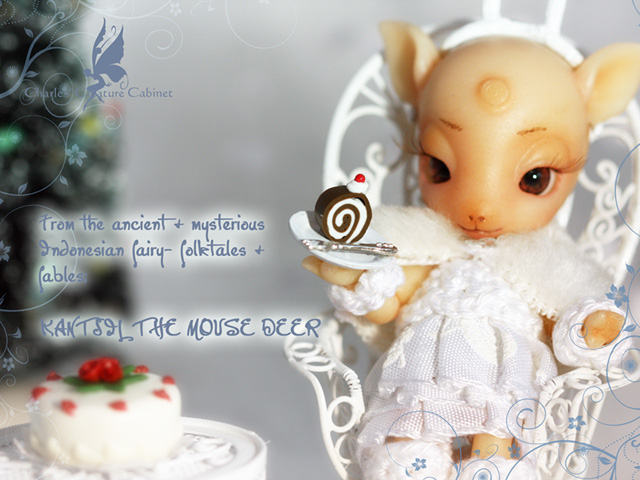In the image, a computer-generated background and a photograph are blended seamlessly. On the right-hand side, a small toy pig, dressed in a white dress, is seated in an ornate, white metallic chair with intricate swirls. The pig holds a plate with a cake and a spoon. Adjacent to this setup, on the left side, a white table holds a white cake adorned with red flowers. The top of the cake displays the inscription: "From the ancient and mysterious Indonesian fairy, folktales and fables, Cancel the Mouse Deer." The floral trellis with blue flowers frames both sides of the scene, adding to the whimsical atmosphere. The upper left corner of the background shows a blurred image of green trees with gray ornamentation, including a fairy and branches. The color palette includes white, gray, blue, tan, brown, red, green, yellow, and pink, enhancing the fairy-tale ambiance of the setting.